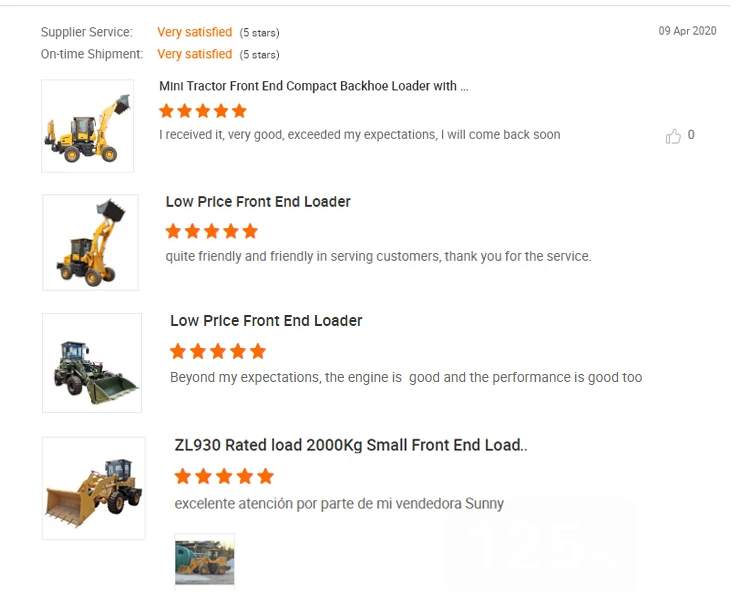The image is a testimonial page from a supplier's website dated April 9, 2020. The page features customer feedback on various machinery, predominantly front-end loaders and compact backhoe loaders. The overall theme highlights high satisfaction, with consistent five-star ratings for supplier service, on-time shipment, and product quality.

1. **Feedback for Mini Tractor and Compact Backhoe Loader:**
   - **Rating:** ★★★★★
   - **Comment:** "I received it in very good condition; it exceeded my expectations. I will come back soon."

   Accompanying the feedback is an image of the mini tractor and compact backhoe loader.

2. **Feedback for Low-Price Front-End Loader:**
   - **Rating:** ★★★★★
   - **Comment:** "Quiet, friendly, and efficient service. Thank you."

   This feedback is accompanied by a photograph of the front-end loader.

3. **Feedback for Another Type of Front-End Loader:**
   - **Rating:** ★★★★★
   - **Comment:** "Low price front-end loader beyond my expectations. The engine and overall performance are excellent."

   The feedback is illustrated with a picture of the specified front-end loader.

4. **Feedback for ZL 930 Small Front-End Loader:**
   - **Rating:** ★★★★★
   - **Comment:** "Rated load 2,000 kg. Excellent attention from the party mini vendor Sunny."

   This feedback also includes a personal image taken by the customer, enhancing the authenticity of their review.

Each piece of feedback underscores the high satisfaction of customers with both the products and services provided by the supplier.